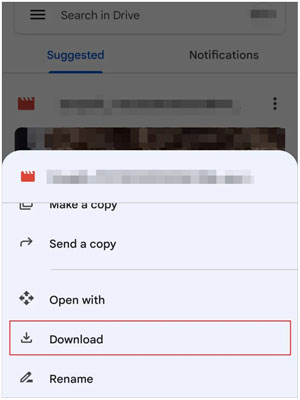The image is a detailed screenshot taken from a smartphone or tablet, identifiable by the unique mobile interface elements. The screen displays a menu typical for managing files or media, heavily resembling an upload interface for YouTube, although certain parts of it are blurred out.

On the left-hand side of the menu, there is a red square adorned with white bands at the top. Adjacent to this square, there is a partially cut-off icon of two overlapping pieces of paper, with the bold text "Make a copy" clearly visible. An arrow pointing to the right accompanies the text "Send a copy."

Below these options, there is an icon resembling a tilting square with four bold black corners, labeled "Open with." Further down, a partially outlined half-square with a downward-pointing arrow and a red rectangle around it is visible, bearing the text "Download."

Continuing, an icon of a pencil with a small adjoining glob, possibly indicating an eraser, is seen, and it is labeled "Rename." 

Circumscribing this menu is a rounded-off square with slightly curved edges. Above this, at the top of the screen, a search bar set against a semi-opaque dark gray overlay is visible. This bar features a settings icon followed by the text "Search in Drive." 

Directly beneath the search bar, two buttons labeled "Suggested" and "Notifications" are visible, with "Suggested" being highlighted in blue and underlined, indicating its selection, while "Notifications" remains in black.

Additionally, there is a section of the image that is blurred out with a red symbol featuring white lines, with another blurred area at the top-right corner of the screen. The detailed graphical elements and careful organization suggest a well-designed file management or media upload interface.